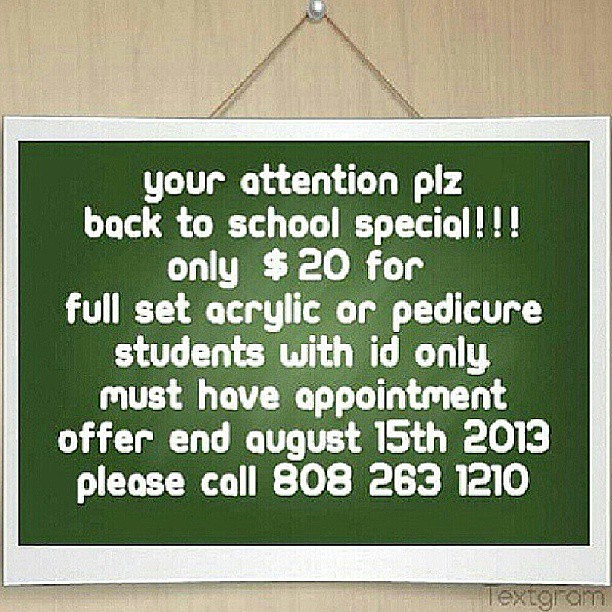The image is a computer-generated advertisement pinned to a light tan door with a silver tack and hanging from a chain. The sign is a white-bordered green rectangle with bold white text, designed to attract attention. It reads: "Your attention please. PLZ. Back to school special!!! Only $20 for full set acrylic or pedicure. Students with ID only. Must have appointment. Offer ends August 15, 2013. Please call 808-263-1210." The text appears to be in a comic sans-like font. At the bottom right corner of the image, there's a watermark that says "Textgram." The photograph is somewhat grainy, indicating a low-quality image.